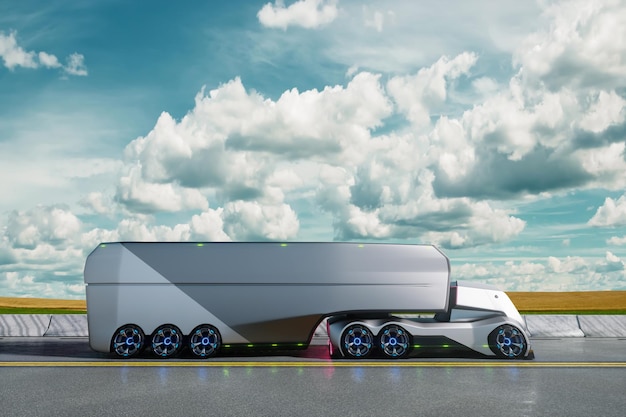This computer-generated image depicts a futuristic electric vehicle, reminiscent of a space-age truck, merging elements of a van and a pickup. The vehicle boasts an unconventional structure with a small, squat cab that looks similar to a Tesla, featuring a bright white front and a predominantly silver rear. The truck has two front wheels and four rear wheels, highlighted by distinctive blue accents along the sides of the tires, although some tires appear oddly deformed. The attached trailer, which arches over the rear of the vehicle, has three wheels at the back and none at the front, giving it an abstract shape akin to an RV.

The setting is a reflective, shiny road marked by a solid yellow center line, with no other vehicles in sight. The background comprises a vast expanse of blue sky filled with clouds, occupying two-thirds of the image, creating a bright, clear day. Additionally, there is a fence composed of wood and marble-like material visible in the scene. Around the vehicle, there are some green and pink lights, adding to the modern, high-tech aesthetic of the scene.